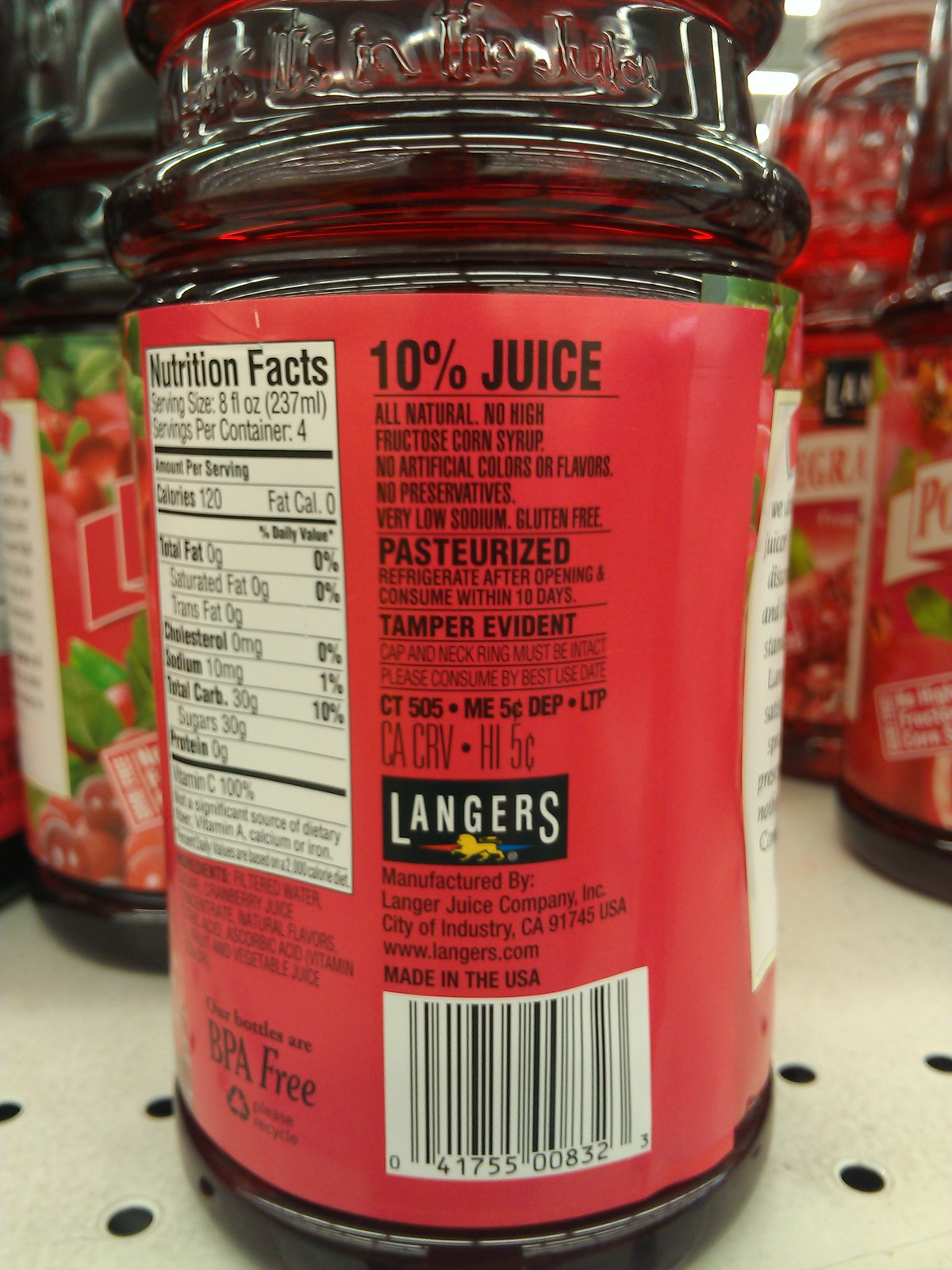On a silver and white shelf, which shows signs of wear with visible scratches and black holes at the bottom, there is a jar prominently displayed. This jar has a plastic lid and is filled with a red liquid. The label on the jar is quite detailed, featuring nutritional information that states each serving size is two-thirds cup, with four servings per container. Each serving contains 120 calories, with total fat, saturated fat, and trans fat all at zero. The jar contains 10 mg of sodium, 30 grams of total carbohydrates, no sugars, and no protein. It states that the product is 10% juice, all-natural, without high fructose corn syrup, artificial colors, flavors, or preservatives. It has very low sodium, is gluten-free, pasteurized, and should be refrigerated after opening. It should be consumed within 10 days of opening. The label further includes a tamper-evident cap disclaimer and mentions a cap and neck seal which must be intact. It intriguingly notes "9.5% MSG glycine" and has various specifications, possibly manufacturing codes and locations: GM HFS USA, CT505, ME 5000, HP, LTP, CACRV, HI 500, alongside mention of being manufactured by the "Lungre Juice Company" in "City of Engineering, California". The company also lists a website, honors.com, and the product is made in the USA.